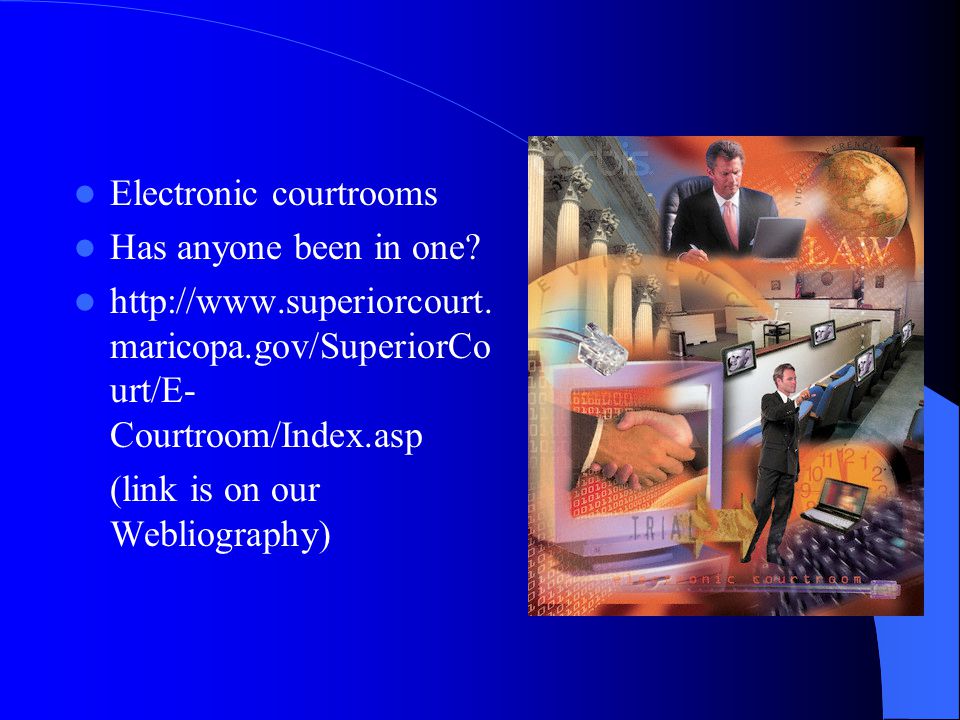This digital image appears to be a detailed slide from a PowerPoint presentation. The background transitions from a bright blue on the left to darker shades on the right, particularly in the upper right corner. On the left side, there are three bullet points in light blue text: 

1. "Electronic courtrooms."
2. "Has anyone been in one?"
3. A website URL: "http://www.superiorcourt.maricopa.gov/superiorcourt/e-courtroom/index.asp," with a note in parentheses stating, "(link is on our Webliography)."

All the text is in white letters.

On the right side of the slide, there is a colorful graphic. At the top of the graphic, an older white man in a red or orange necktie sits in front of a gray laptop, appearing slightly confused. This man is centered and right-aligned. Above him, there is a golden globe icon with the word 'LAW' beneath it. Further details in the image include a computer monitor on the lower left displaying two hands shaking, both individuals appear to be wearing suits. Additionally, the lower right corner features a faded image of a clock and another man in a suit pointing at something. The color palette of the slide includes blue, white, dark blue, black, red, orange, yellow, and brown, emphasizing the professional and educational nature of the content.